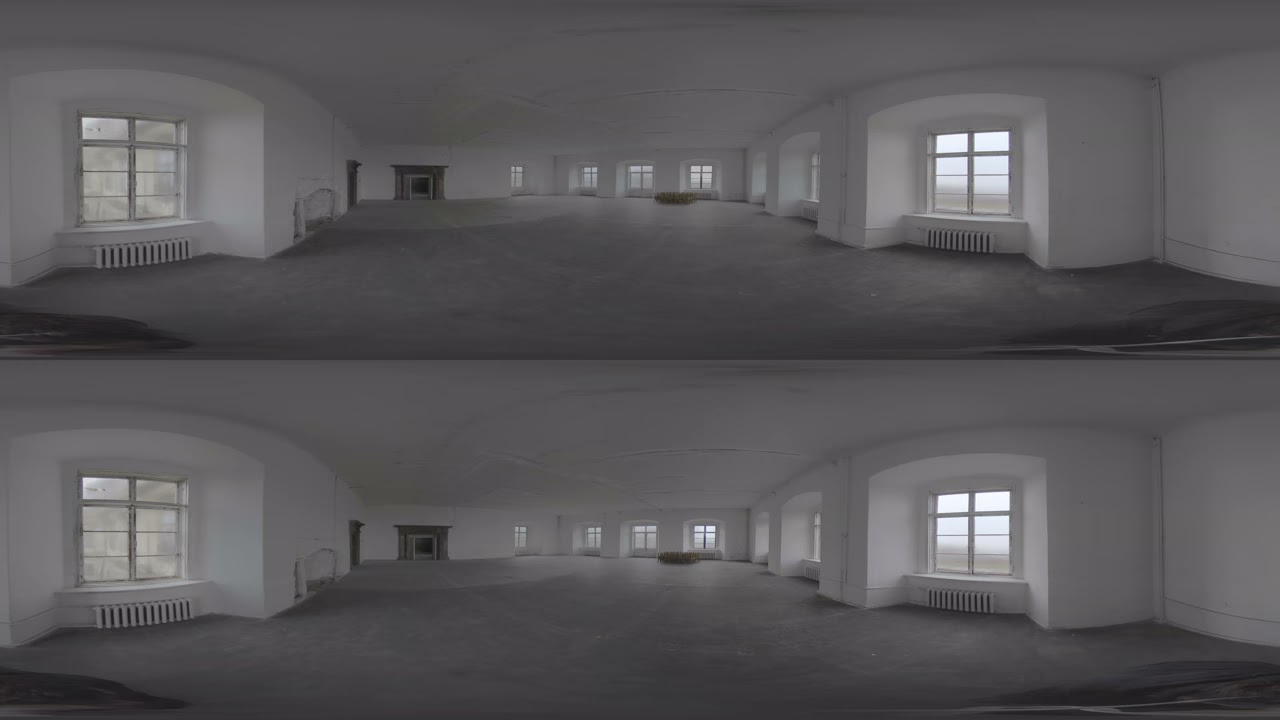The picture consists of two identical grayscale images stacked one above the other, each depicting a large, open interior space, possibly of a home or office. The flooring is a darker shade of gray, contrasting with the all-white walls and ceiling. On the left side of the room, a double window with a radiator beneath it opens the space. Moving right, the room extends and deepens, revealing a fireplace on the far wall. There are four windows in the background and three more windows on the right wall, each with radiators beneath them, tucked into alcoves that create built-in seating sills. The windows are framed by subtle archways, adding an architectural interest to the space. The images, although grayscale, hint at some color outside the windows, but the interior details remain the focus, showcasing the wide, open, and symmetrical layout of the room.